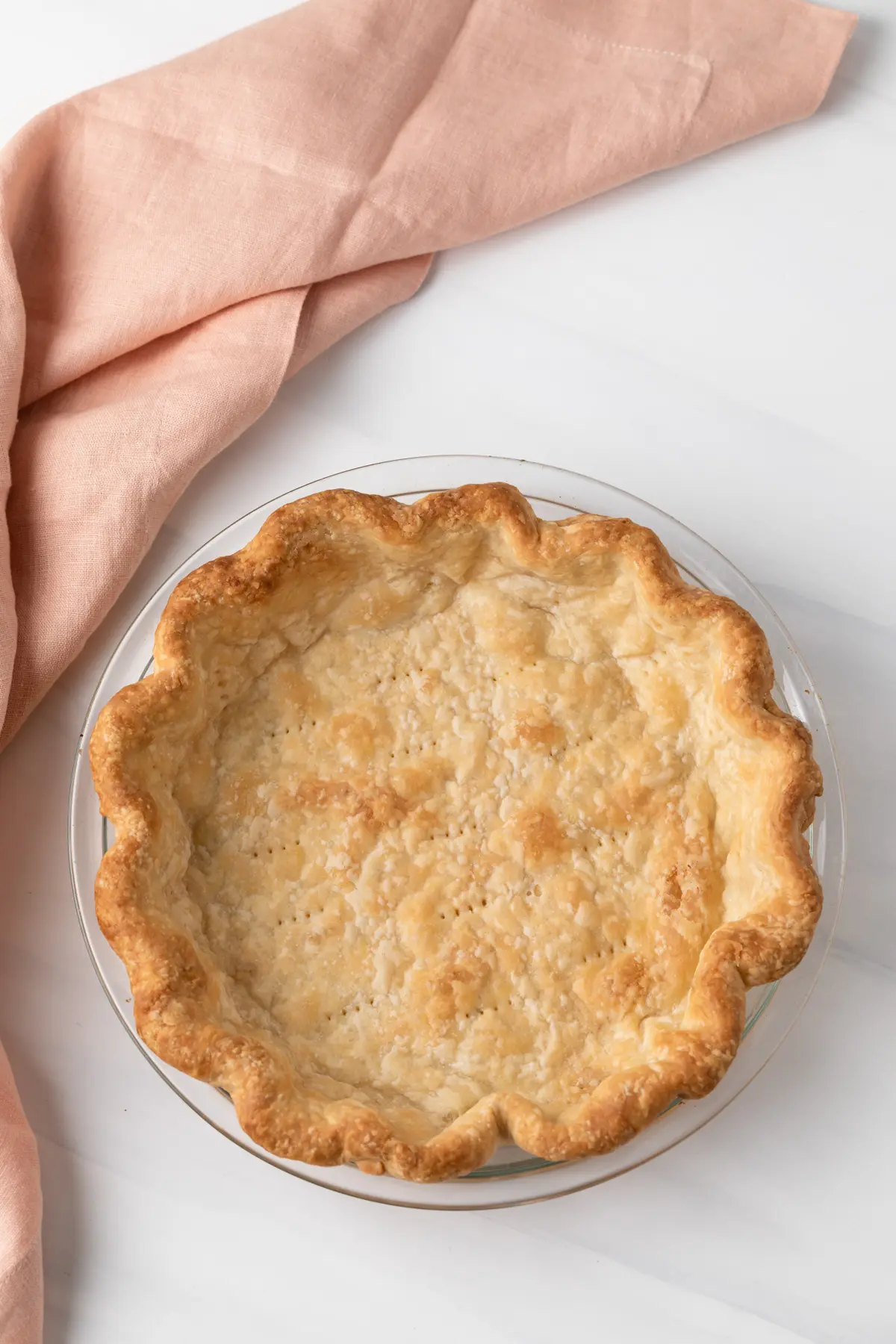This is a detailed photograph depicting a golden brown, handmade pie crust resting on a white plate with a thin gold border. The pie is viewed from directly above, showcasing its wavy, thick crust with a darker brown edge. The crust bears a textured middle with multiple fork-punched holes: four on the left, five down the center, and four on the right. The plate sits on a white table, accompanied by a pinkish-peach cloth napkin that is visible at the top and along the left edge of the image.